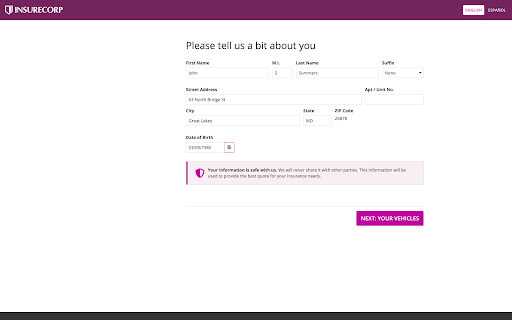In a user interface for Slurbicorp, the screen prompts the user with "Please tell us a bit about you," positioned at the top-center. Below this prompt, a graphic design element featuring a half white, half pink shield, with a vertical pink line adjacent to it, is displayed. The screen is adorned with various placeholder texts, represented by repeated "blur" entries, which likely indicate areas for user input or labels that are yet to be finalized or translated.

Towards the mid-section of the screen, a horizontal grey line separates the top sections from the user action area. Here, a pink button labeled "Next, Your Vehicles" appears, suggesting the next step in the user process. The top-right corner of the screen contains additional placeholder text ("blur blur"), all set against a maroon background. The central part of the screen maintains a clean, white background to emphasize clarity and focus. Finally, at the very bottom, a black horizontal line spans the width of the interface, providing a visual boundary and structural balance.